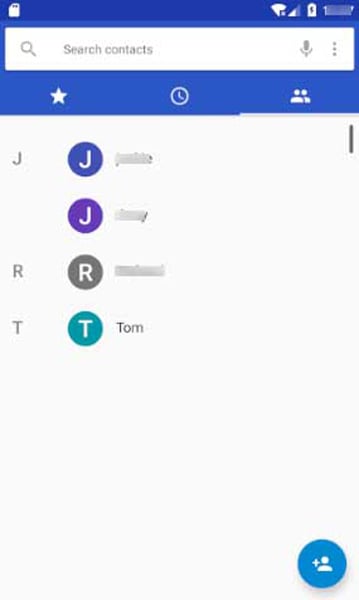In this image of a mobile device's contact page, several elements and information are partially obscured or blurred for privacy. 

At the top of the screen, a dark navy blue border holds essential status icons. On the upper left, a small white SIM card icon is displayed. The upper right corner houses a cluster of indicators: a Wi-Fi icon with an adjacent 'X' suggesting an incomplete signal, a data icon that's half full, a fully charged battery icon featuring a lightning bolt, and a smudged-out section obscuring additional details.

Below the status bar, there is a search bar labeled "Search contacts" which includes a microphone icon for voice search functionality.

A navigation menu features selectable options for "Favorites," "People," and "Recent," displayed with corresponding icons of a star, a person, and a clock. The "People" tab is currently selected.

Contacts are listed with circular profile images and initials. The first contact is represented by a blueish-purple circle with the initial "J." The second contact has a violet-purple circle, also with the initial "J." Both of these entries are heavily smudged to conceal further information. Additional contacts include one with a gray circle labeled "R" and a blueish-green circle labeled "T," with the name "Tom" accompanying the latter. The remaining contact details are also smudged.

Overall, the image captures the essential layout and functions of the contact page while ensuring privacy by obscuring sensitive information.